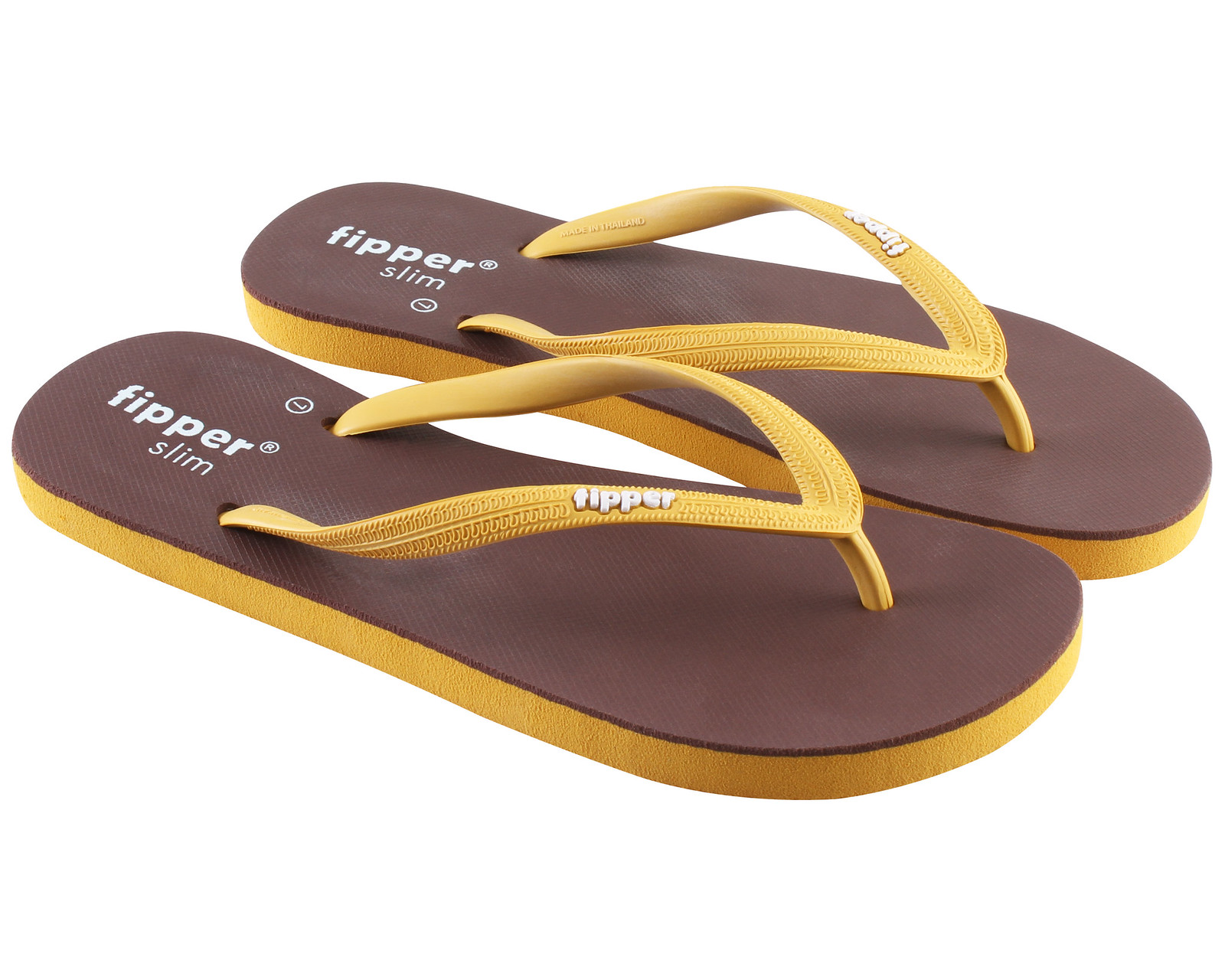This detailed close-up photograph features a pair of flip-flops with distinctive design elements. The flip-flops have yellow straps with a grooved, tire-like texture for added grip and comfort. These straps are marked with the brand name "Flipper" in raised white text. The sole is a combination of brown and mustard-yellow foam, providing a cushioned base for the feet. On the brown part of the sole, near the heel area, the words "Flipper Slim" are printed in white, accompanied by a registered symbol. Additionally, there's a size indicator—'L' in a circle—denoting size 7. The yellow underside matches the color of the straps, creating a cohesive design. The flip-flops are constructed from a foamy material, further enhancing their lightweight and comfortable feel.